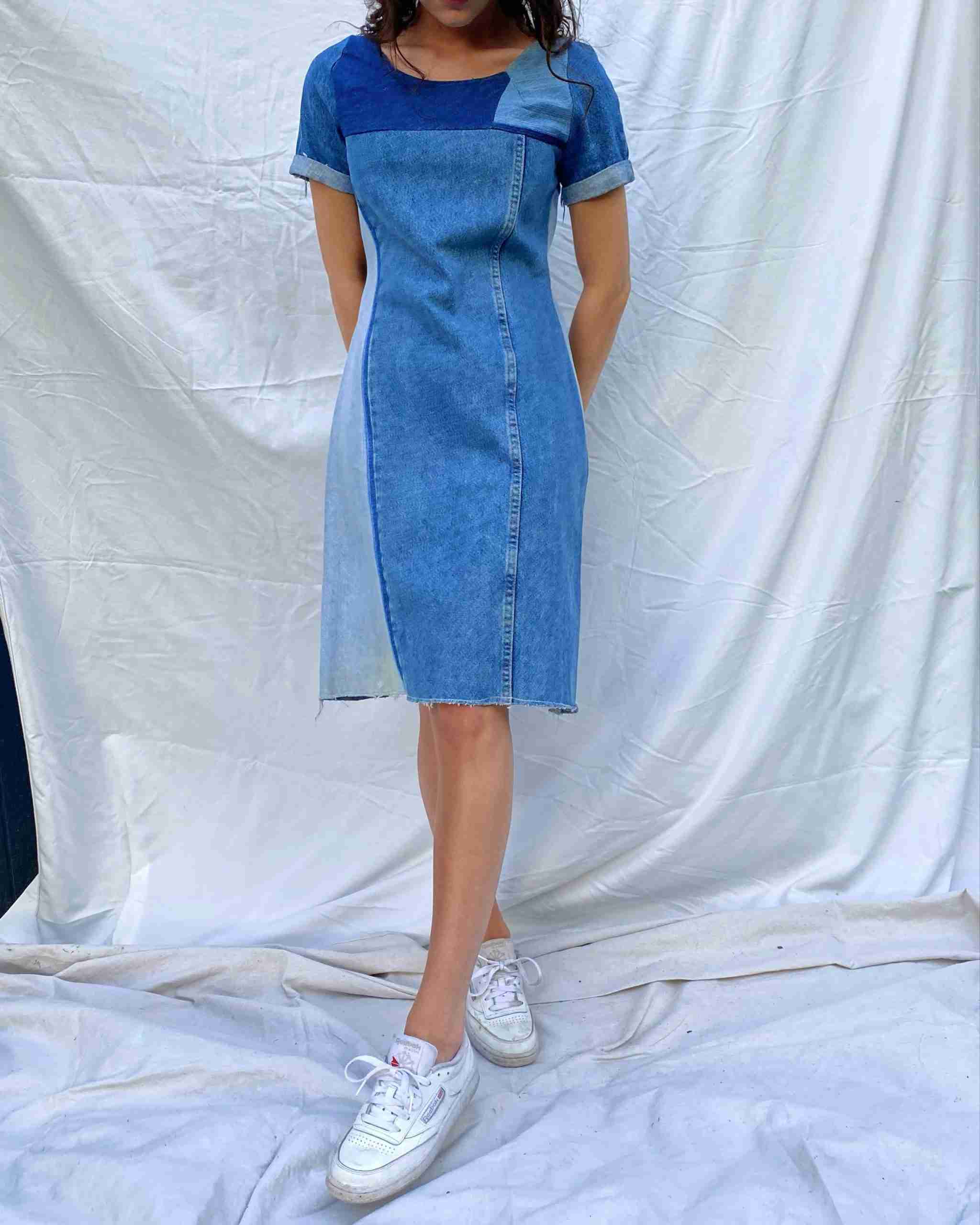A photograph features a woman standing with her hands behind her back and her left leg crossed in front of her right. She has a light, slightly tanned complexion and is dressed in a unique blue denim dress composed of various panels stitched together, showcasing different shades of blue. She is not wearing any pants or leggings, and her outfit is complemented by slightly distressed white shoes. The image is cropped so her face is not visible. She stands against a plain backdrop fashioned from a white bedsheet, which also extends beneath her, obscuring the floor. The time of day the photograph was taken remains indeterminate.